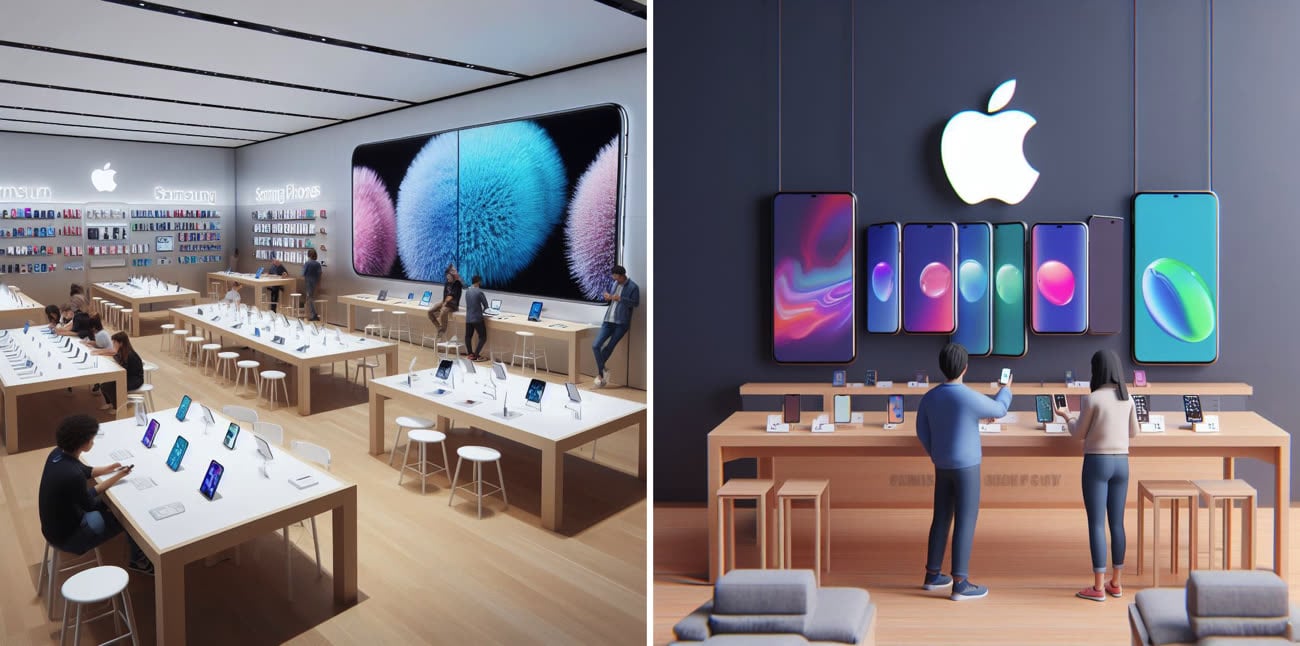The image presents two digitally rendered scenes of Apple stores side by side, each featuring realistic human figures and a variety of Apple products. 

In the left image, the store interior is modern and well-lit, characterized by sleek tables with stools positioned in front of them. These tables display various Apple devices, including phones and tablets. Mounted on the right wall are two large screens, and a glowing Apple symbol decorates the farthest wall, adding a signature touch to the store’s ambiance. The store is bustling with activity, as eight individuals are seen interacting with the devices at the tables.

The right image depicts a simpler scene with two people, a man and a woman, standing in front of a table set against the wall. A secondary table, placed between them and the wall, displays an assortment of Apple products they are examining. Two gray chairs are situated nearby, adding to the store’s functional decor. The background features a display of decorative Apple phones, along with another prominently lit Apple symbol.

Overall, both images capture the essence of a typical Apple store, highlighting the clean, minimalist design and the interactive experience for customers.